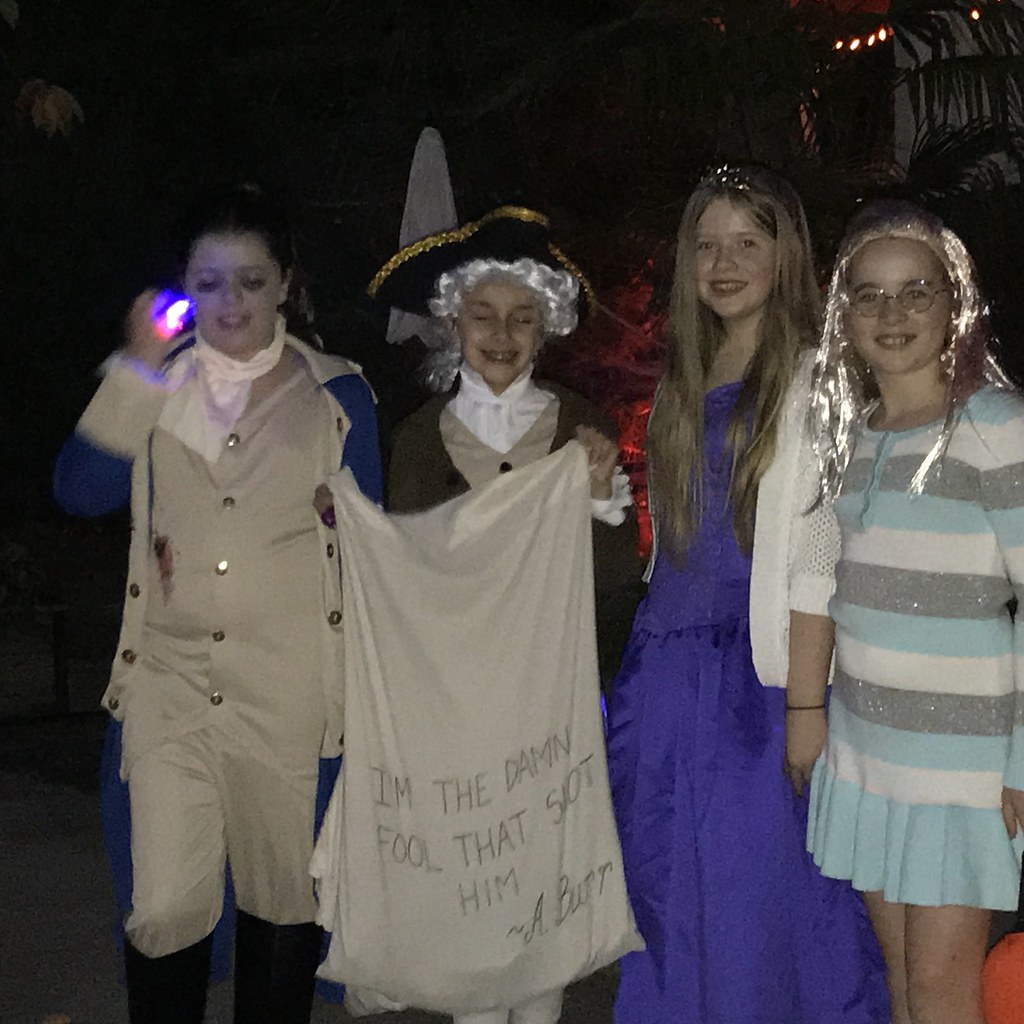The image portrays four children, approximately 10 to 16 years old, dressed in elaborate costumes. From left to right, the first child, whose gender is indistinguishable, is dressed in an 18th-century style outfit, complete with a white costume wig, a black pirate hat trimmed in gold, a white shirt with a high collar, a beige vest, a brown jacket, and black knee-high boots. They hold a large beige pillowcase with the inscription, "I'm the damn fool that shot him. A. Burr," suggesting an Aaron Burr costume.

The second child, a girl with long, light brown hair, is wearing a blue satin-like dress accompanied by a white sweater. She appears to have a small shiny tiara in her hair, adding to her regal appearance.

The third child, a girl with a shiny gold wig and gold-rimmed glasses, wears a distinctive sweater dress with white, gray, and turquoise stripes that transition into a turquoise ruffle at the bottom. 

Lastly, the fourth child, a girl with her hair tied back, dons an ensemble consisting of a white shirt, a beige one-piece outfit with long sleeves that might be pants, a blue jacket, and black knee-high boots. She holds a shiny object in her right hand, although it's partially blurred in the image. The background appears to be dark, indicating that the photo was likely taken at night, possibly during Halloween festivities.